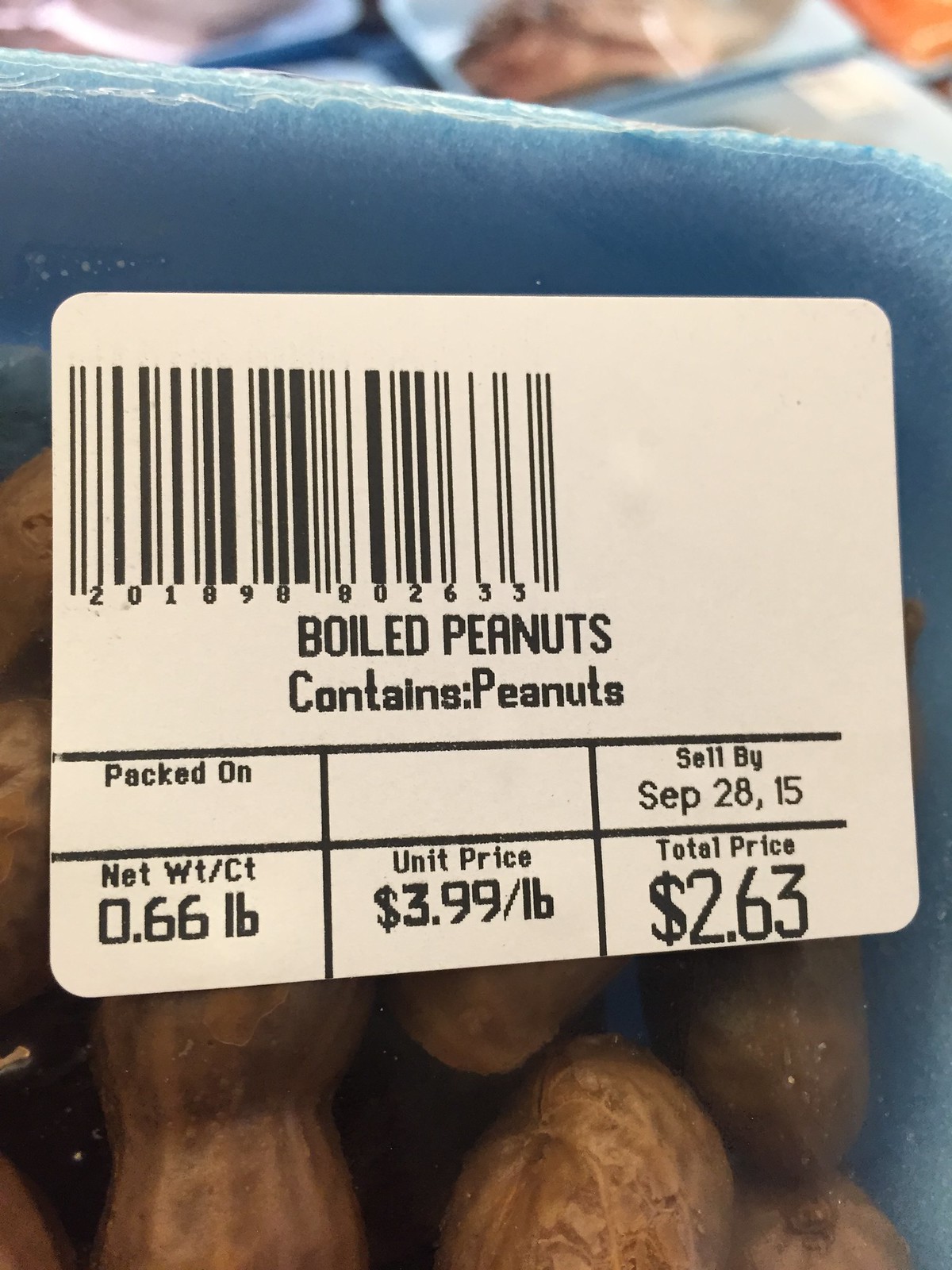This close-up photograph captures a product label from a grocery store adhered to a plastic-wrapped foam container of boiled peanuts. The label prominently features a barcode and the title "Boiled Peanuts." Beneath the title, there's an allergy notice stating "Contains Peanuts," along with product specifications such as a net weight of 0.66 pounds. The unit price is listed as $3.99 per pound, resulting in a total price of $2.63 for this package. The label also indicates a sell-by date of September 28, 2015. The container is blue, and the boiled peanuts inside are visible, characterized by their brown color and slightly altered texture due to the boiling process. In the background, the out-of-focus shapes of additional grocery store products can be seen, adding context to the setting.